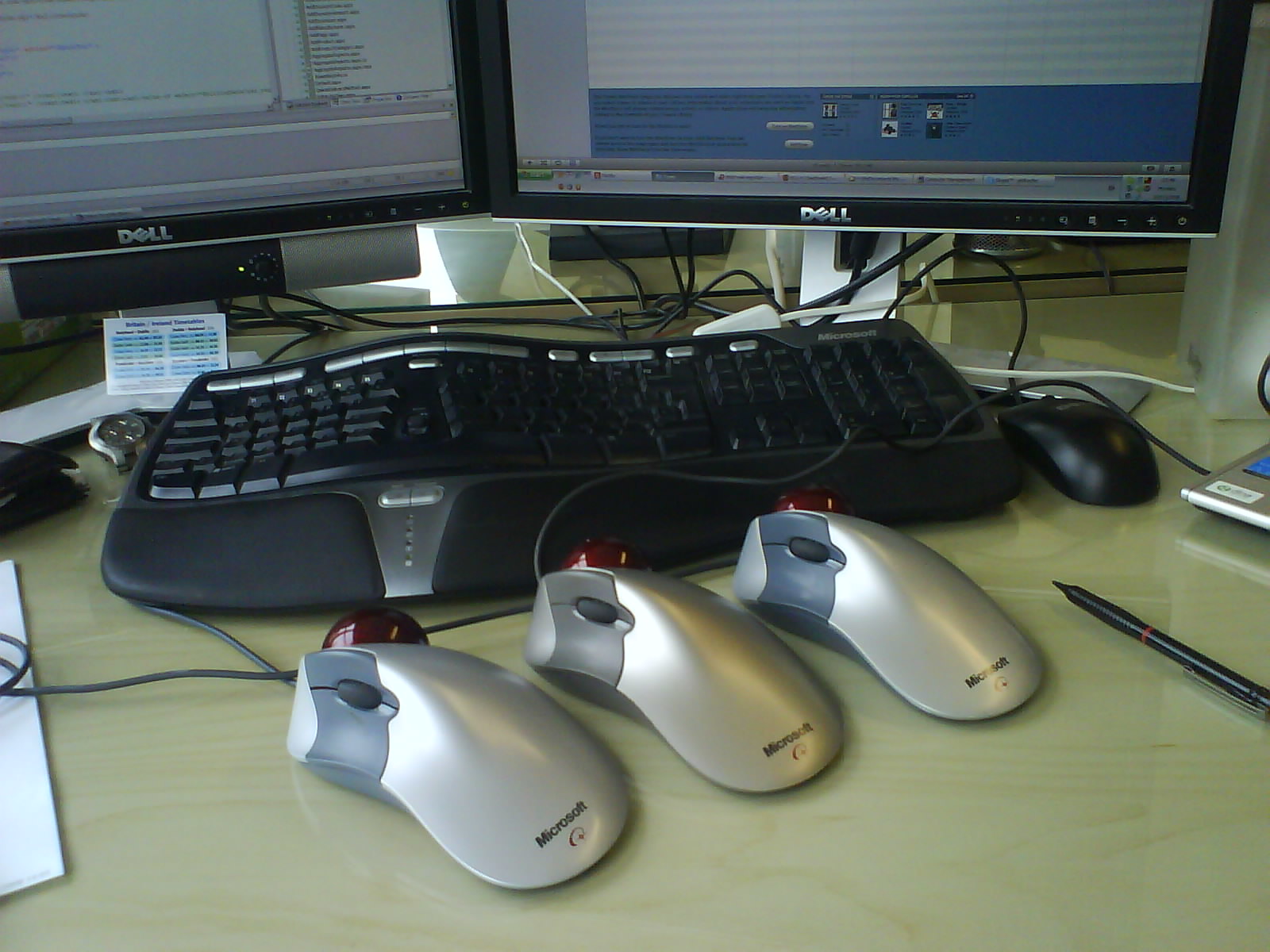This color photograph captures a detailed view of a computer workstation. Dominating the top third of the image are two large Dell monitors, positioned side by side and featuring black frames with the Dell logo in silver at the bottom. One screen displays what appears to be a white-painted brick wall with a blue stripe and a small cartoon figure at the base, while the other shows what looks like an Excel spreadsheet. Below the monitors, the desk surface is organized but busy. 

At the center, there is a sleek black ergonomic keyboard, notable for its curved design, which purportedly aids in wrist comfort during extended typing sessions. Adjacent to the keyboard sits a matching black mouse. In the foreground, three silver and gray Microsoft ergonomic mice are prominently displayed. These mice have distinctive red trackballs, intended to ease hand strain through ergonomics. Additionally, a stylus and the edge of a laptop are visible to the right, further contributing to the tech-centric environment. Various wires appear to be well-organized, connecting the peripherals seamlessly to the workspace setup.